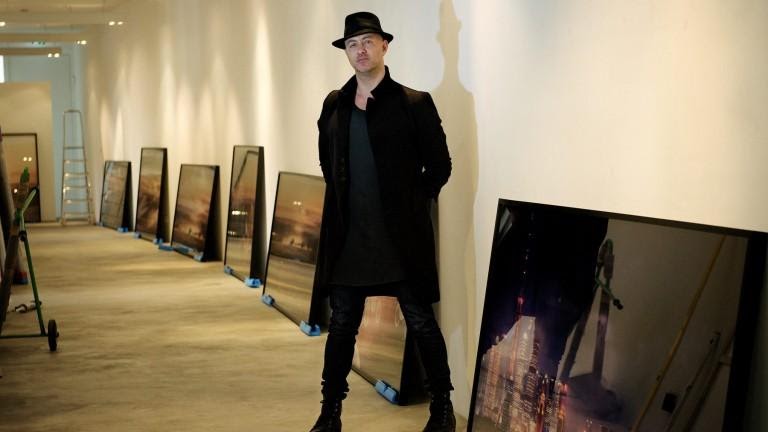This photo captures the interior of a well-lit, photorealistic room or long hallway with a distinctive art gallery vibe. The central focus is a Caucasian man, facing the camera, dressed entirely in black: a black hat with a rim reminiscent of the 1940s, a long black coat, a black shirt, tight black pants that gather at his black boots, creating a slightly layered effect. With both hands in his pockets, he stands confidently on a tan, mottled floor. 

Behind him, the white wall stretches into the background on the left side, receding from the foreground towards the left. Leaning against this wall are several framed photographs or paintings of varying sizes, though glare makes it difficult to discern most of their subjects. The closest artwork, a cityscape at night, is vividly visible. 

Further down the hallway, a silver stepladder is positioned against the wall, and nearby, various items, including a small dolly with wheels, rest on the floor. Despite the room's shadows and varying lighting, the overall atmosphere is clean and organized, highlighting the intriguing blend of modern and classic elements.